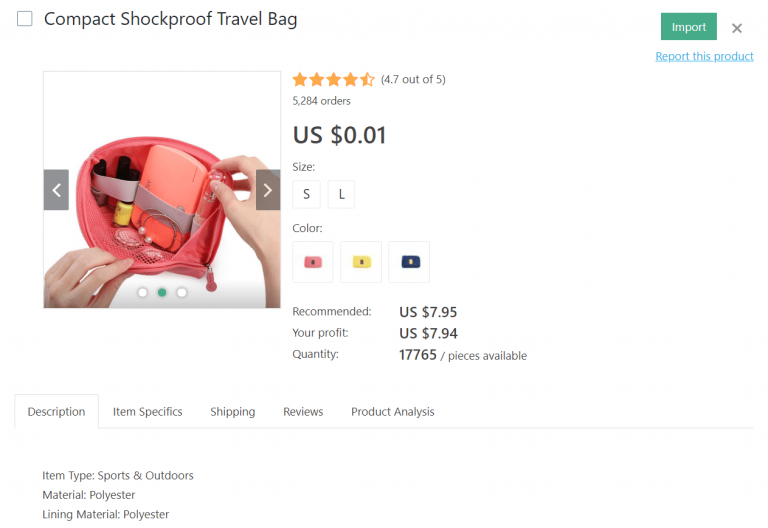**Compact Shockproof Travel Bag for Sale**

This detailed image showcases a Compact Shockproof Travel Bag available for purchase. 

- **Top Left Corner**: The image features an unchecked checkbox and the caption "Compact Shockproof Travel Bag."
- **The Bag**:
  - The bag is displayed in an open position, revealing its vibrant orange-pink hue.
  - Inside, various items are arranged to demonstrate the bag's capacity and organizational features. A mesh pocket and a couple of straps are visible, holding the items securely in place.
  - A person's hands are shown handling the bag, indicating ease of use.

- **Additional Details**:
  - Star Rating: 4.7 out of 5 stars
  - Number of Orders: 5,284
  - Price: $0.01 (U.S. dollars)
  - Available Sizes: Small and Large
  - Available Colors: Orange-Pink, Yellow, and Dark Blue (or possibly Black)
  - Additional Pricing Information: Recommended Price - $7.95, Potential Profit - $7.94
  - Stock Quantity: 17,765 pieces available

- **Tabs and Descriptions**:
  - The page features five tabs running across: Description (highlighted), Item Specifics, Shipping, Reviews, and Product Analysis.
  - Under the "Description" tab, the item details read as follows:
    - **Item Type**: Sports and Outdoors
    - **Material**: Polyester
    - **Lining Material**: Polyester

This caption provides an extensive overview of the travel bag, highlighting its features, specifications, and available options for potential buyers.